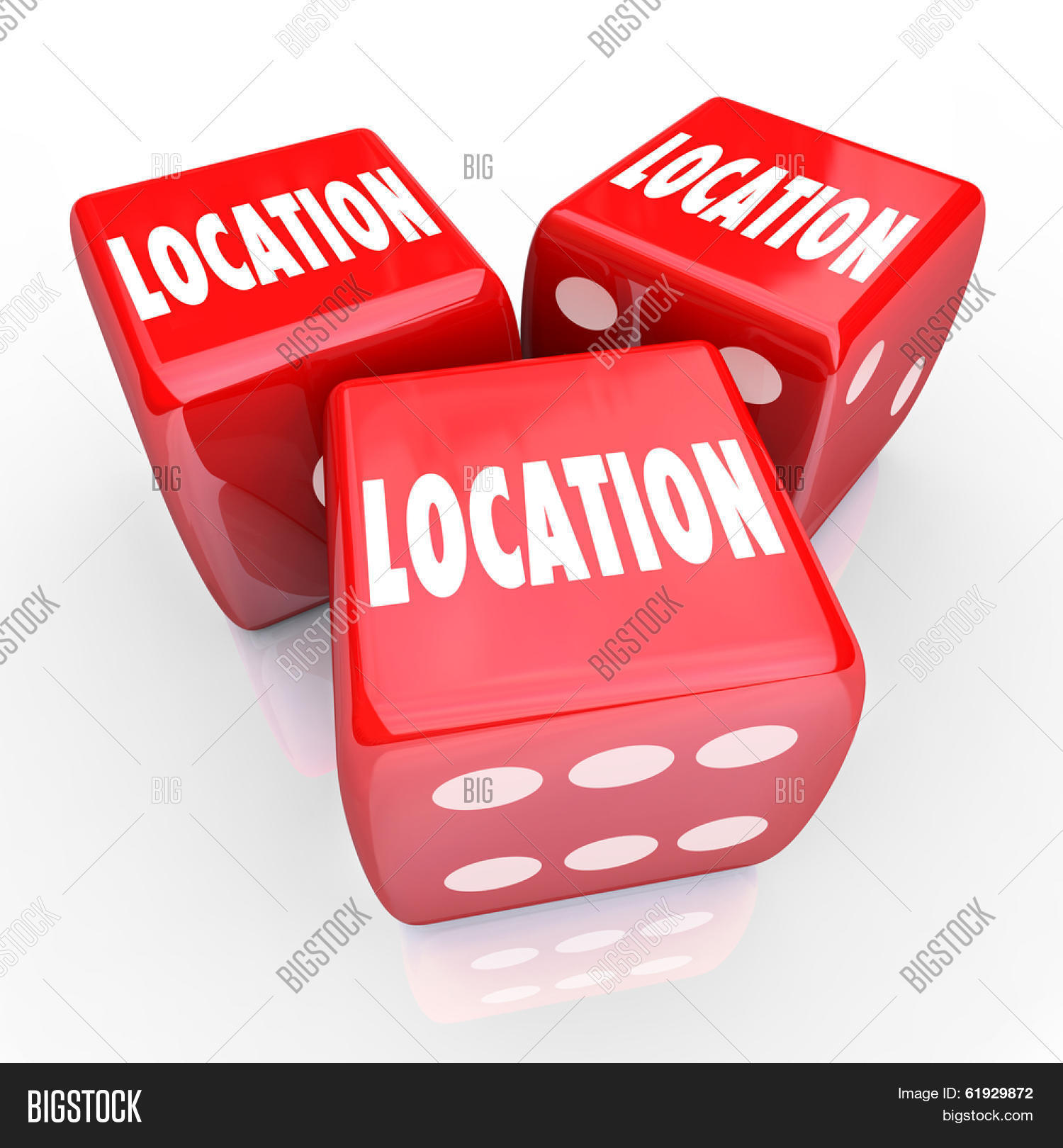The image is a detailed 3D rendering of three large, red dice, each with white pips on their faces. On the top-facing side of each die, the word "location" is prominently displayed in white, replacing the usual numbers. The dice are positioned on a highly reflective surface, creating a mirror-like effect that showcases their reflections beneath them. Specifically, the bottom-most die shows six pips on its underside, the top-left die displays one pip, and the top-right die has four pips on the bottom and two pips on the right. Overlaying the entire image is a repeating semi-transparent gray watermark that reads "big stock" in diamond-shaped patterns. This image's elements suggest a thematic emphasis on the significance of location, possibly targeting real estate or related fields.